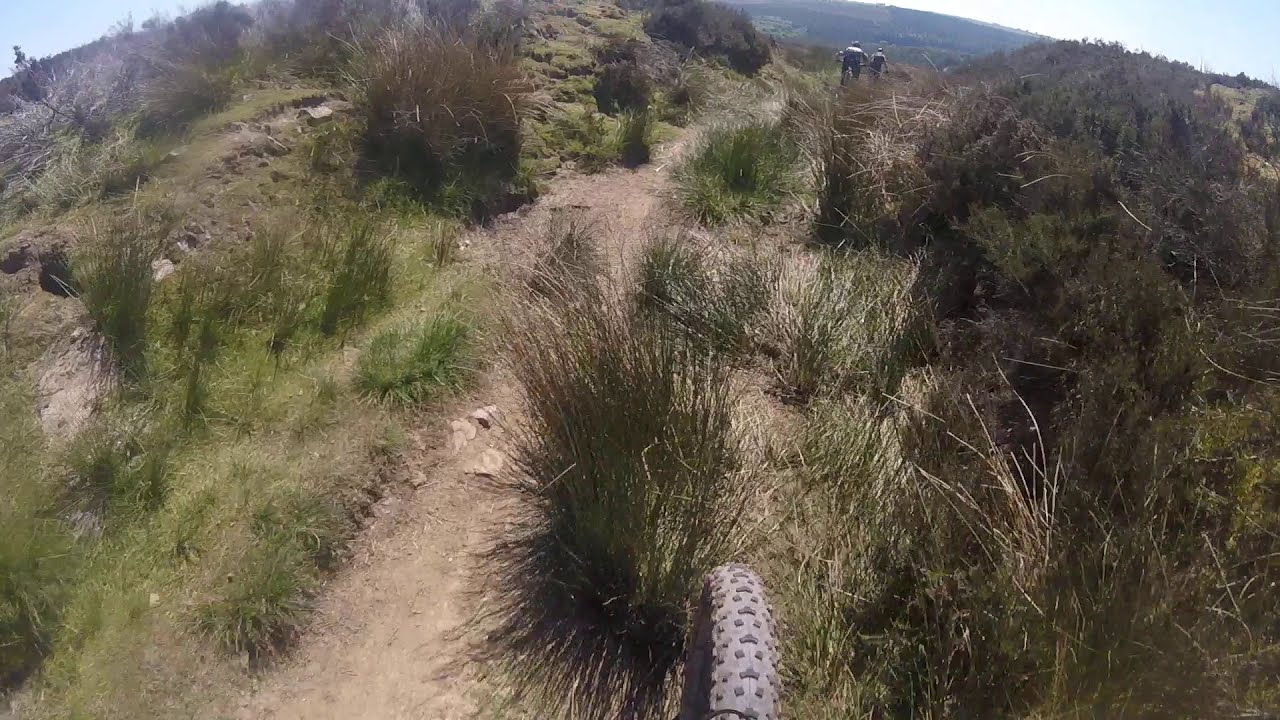Looking down what appears to be a rugged mountain bike trail, the bottom center of the photograph, slightly to the right, reveals the deep-treaded, spiky front tire of a mountain bike, suggesting an off-road adventure. The winding dirt path, slightly to the left and overgrown with spiky green brush and varied grasses, leads the eye upward toward the top right of the image, where two distant mountain bike riders are visible. The terrain is dry and sandy, dotted with hardy green plants, possibly sage, hinting at an arid, western U.S. setting. The area is hilly and mountainous, with hints of granite rising next to the trail, and small patches of blue sky visible at the photo's edges. The image, likely captured with a wide-angle lens, possibly from a GoPro mounted on the rider's head, showcases the challenging yet picturesque trail as it curves and climbs through the rugged landscape.